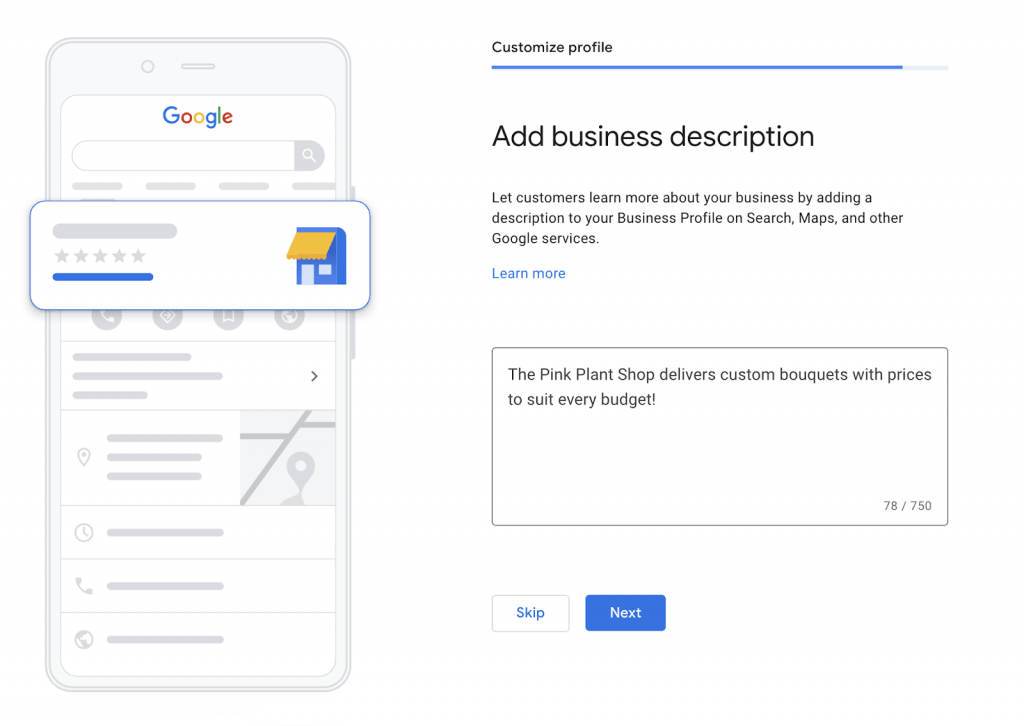The image features a large smartphone screen displaying a Google business profile setup interface. At the top of the screen, there is a gray oval with five gray stars beneath it, indicating a rating system. The main focus is a Google search bar accompanied by various gray rectangles representing placeholder text.

Additionally, there is an illustrated blue building with a yellow canopy, likely representing a shop icon. On the right side, a message prompts users to "Customize Profile" and provides a detailed business description area encouraging businesses to add a description for better visibility on Google Search, Maps, and other services.

A section below contains text that introduces "The Pink Plant Shop," which offers custom bouquets at prices suitable for various budgets, with a progress tracker showing "$78 out of $750". Below this section, there is a "Learn More" link in blue text, alongside a "Skip" option.

At the bottom, a blue rectangle with white text states "Next." This entire interface is part of setting up a Google business profile website.